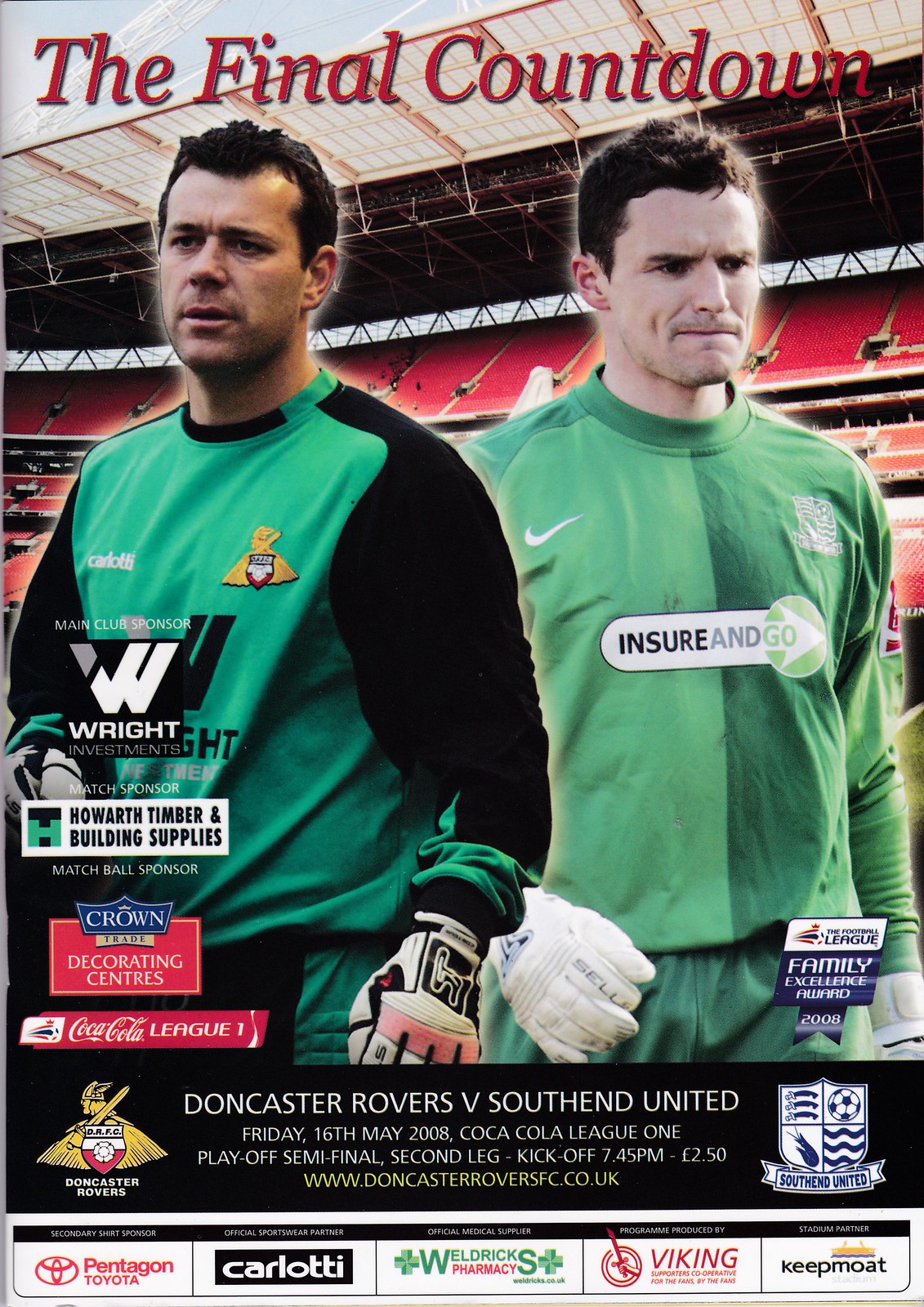This image is an advertisement for a soccer game, prominently featuring an event titled "The Final Countdown" in bold red letters across the top. In the center, two soccer players stand shoulder to shoulder, gazing into the distance. To the left, the player has very fair white skin, short black hair, and is dressed in a green long-sleeved shirt, featuring a Nike logo, green shorts, and white gloves. The player on the right appears slightly darker and heavier, also clad in a green long-sleeved shirt with black sleeves, green shorts, and white gloves. 

Behind them is an empty soccer stadium with red seats, setting the scene for the event. The text beneath the image reads "Doncaster Rovers vs. Southend United, Friday, 16th of May, 2008, Coca-Cola League One, Playoff Semifinal, Second Leg, Kickoff 7.45pm," followed by the price "$2.50" and the website "www.doncasterrovers.co.uk."

The advertisement is peppered with numerous sponsorship logos at the bottom, including Pentagon Toyota, Carlotti, Weldrick's Pharmacy, Viking, and Keep Moat, as well as additional sponsors like Riot Investments, Howard's Timber and Building Supplies, Crown Decorating Centres, Coca-Cola League, and Doncaster Rovers. This detailed visual serves to promote the pivotal match, building anticipation among fans of the Doncaster Rovers football club.